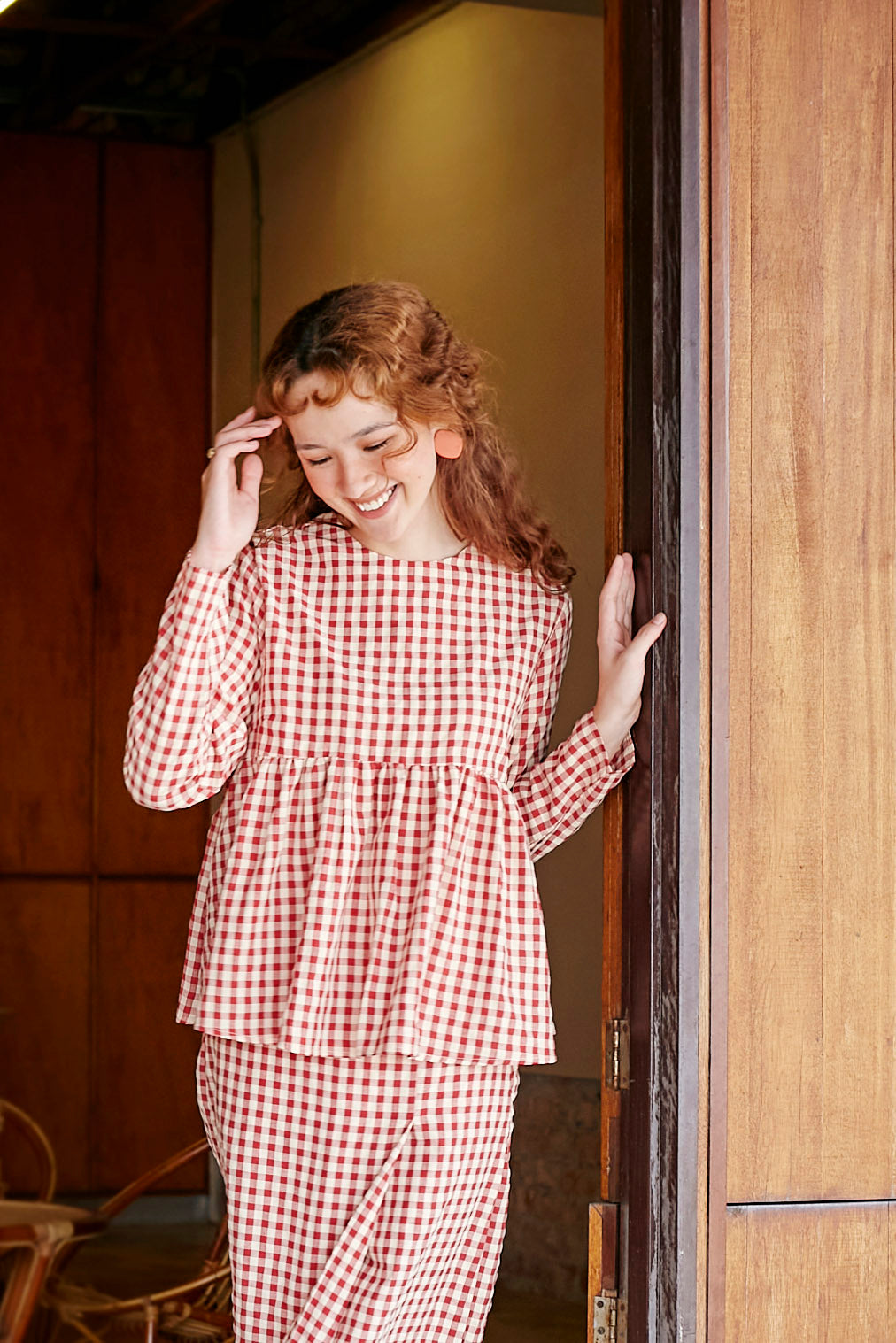This color photograph, in portrait orientation, portrays a young woman, approximately 18 years old, with long, curly red hair, standing in an open doorway. The door takes up the left two-thirds of the image. She is centered slightly to the left, framed from the top of her head to about mid-knee. The woman wears a coordinated two-piece outfit consisting of a short bodice top and a flouncy wraparound skirt, both featuring a small red and white checkered pattern. Her long-sleeved top and matching skirt exude a casual yet stylish vibe, reminiscent of modern fashion photography with a focus on realism. 

The young woman smiles warmly, looking down with her eyes closed, her teeth showing slightly. She wears large, round peach-colored disc earrings. Her left hand rests on the doorframe, while her right hand touches her brow, as if adjusting her hair or shielding her eyes. Behind her, the room features gold walls and some chairs, contributing to the cozy, inviting atmosphere. The ambient light, seemingly soft and overcast, illuminates her from the front, highlighting her lively expression and vibrant hair.